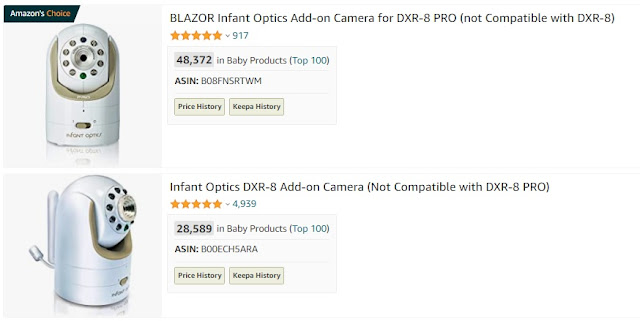This image appears to be a screenshot from an Amazon product page featuring baby monitoring devices. In the upper left corner, a blue or black banner indicates "Amazon’s Choice." The image showcases two similar products that are white and oval-shaped, resembling small robots with dots around the perimeter and a prominent circle in the center. Each device has a cord extending from it, presumably for power or connection purposes.

The first product description reads "Blazer Infant Optics Add-On Camera for DXR-8 Pro, not compatible with DXR-8," and is highly rated with five stars. The second product, also an add-on camera, is labeled "Infant Optics DXR-8 Add-On Camera, not compatible with DXR-8 Pro," and it too boasts a five-star rating. Although the image does not display prices, it is clear that both products are designed for use as baby monitors and are part of the Infant Optics brand lineup.